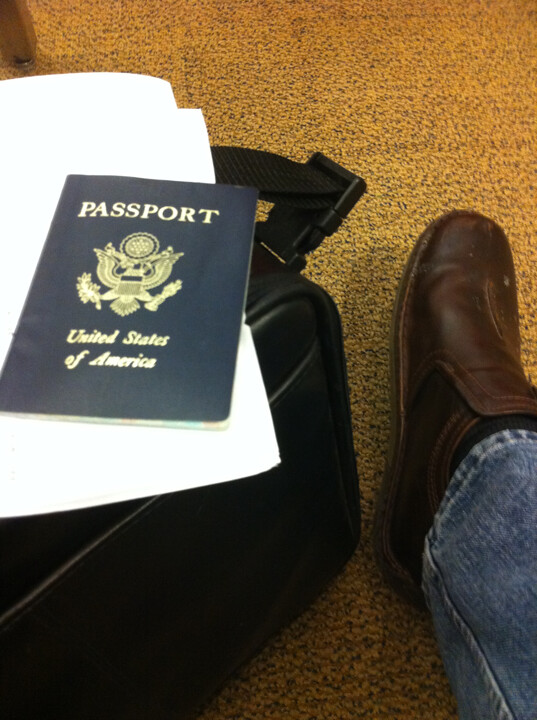The photograph, taken from a seated perspective, captures various items on an orange carpet speckled with black. On the left side of the image, a black travel bag with a visible strap rests on the floor. On top of this bag lies a white folder, and prominently displayed on the folder is a blue American passport. The passport cover features gold lettering that reads "Passport" and "United States of America" above and below the Great Seal of the United States, which depicts an eagle holding olive branches and arrows in its talons. To the right side of the image, a brown loafer-style shoe is visible, partially concealing a green sock and some black socks tucked inside. Emerging from the shoe is the bottom segment of a pant leg made of blue denim. The photograph’s background and focal objects together evoke a sense of casual travel.